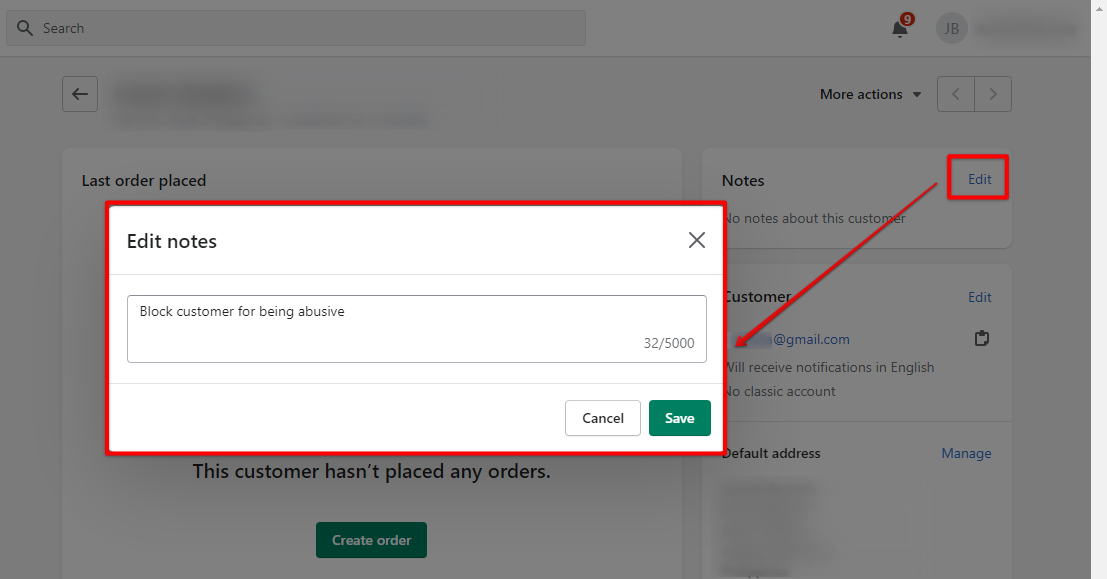The image is a detailed screenshot of a web interface featuring a dialogue box titled "Edit Notes" located at the top left corner. Directly below this title, there is a text box containing the message "Block customer for being abusive." At the bottom right of the text box, it displays a character count, showing "32 out of 5,000," indicating the number of characters used and the total character limit. Additionally, there are two actionable buttons beneath the text box. The button on the left is labeled "Cancel," while the button on the right is labeled "Save," which is highlighted in a forest green color.